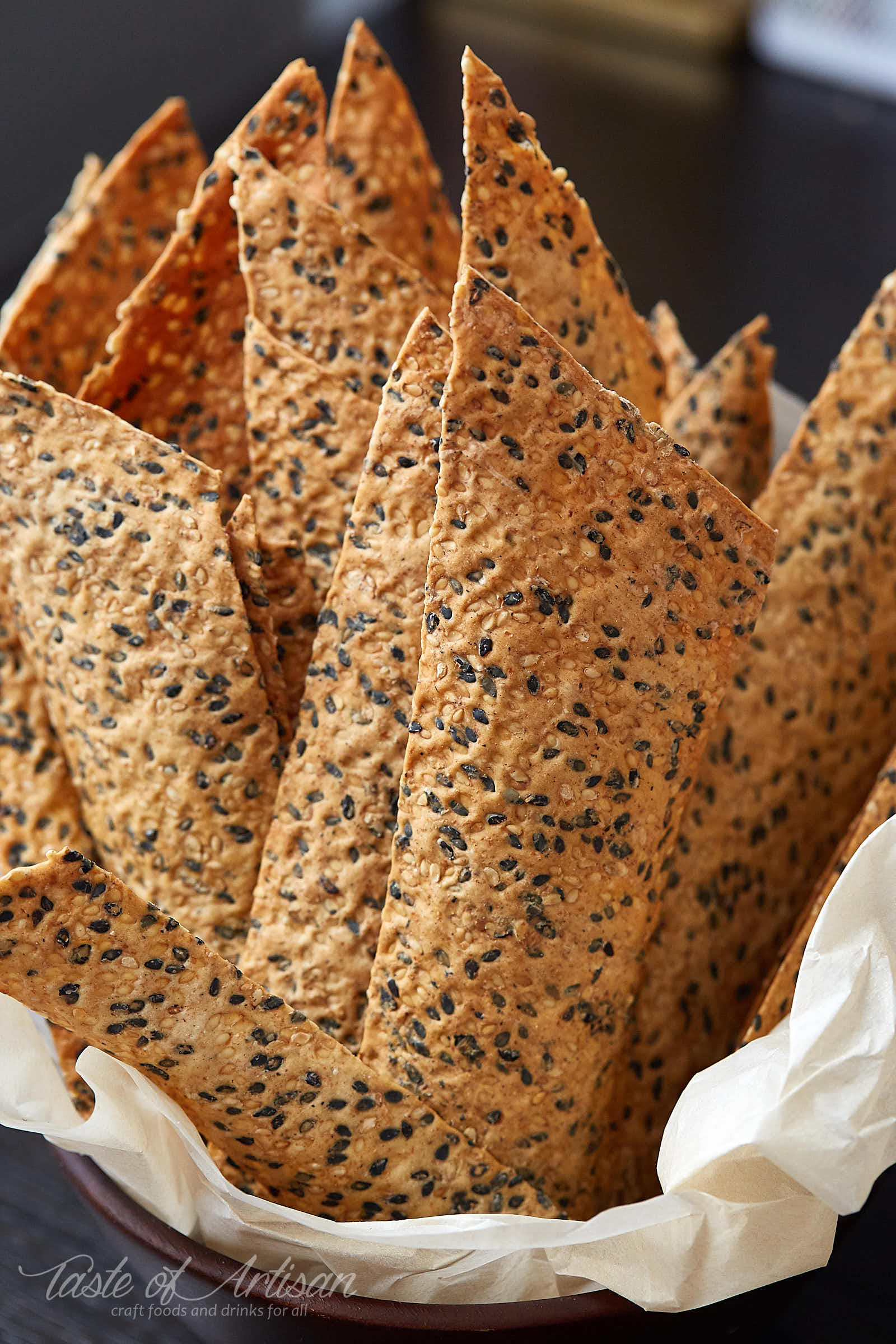This detailed, color photograph captures an up-close view of food presented in an earthy brown, brass-looking basket. The basket is lined with a crumpled white cloth or napkin that provides a crisp contrast to the contents. Resting within, there are approximately 16 to 17 brownish-orange, dry-looking nacho-like strips, which are notably larger and longer than typical nacho chips. Each strip is generously embedded with a mix of black and white sesame seeds, giving them a heavily seeded appearance. The lower bottom left corner of the image features a somewhat transparent cursive watermark that reads "Taste of Artisan," followed by the printed phrase in small, white letters, "Craft Foods and Drinks for All." The background hints at a dark, possibly marble countertop, adding to the artisanal aesthetic of the scene.